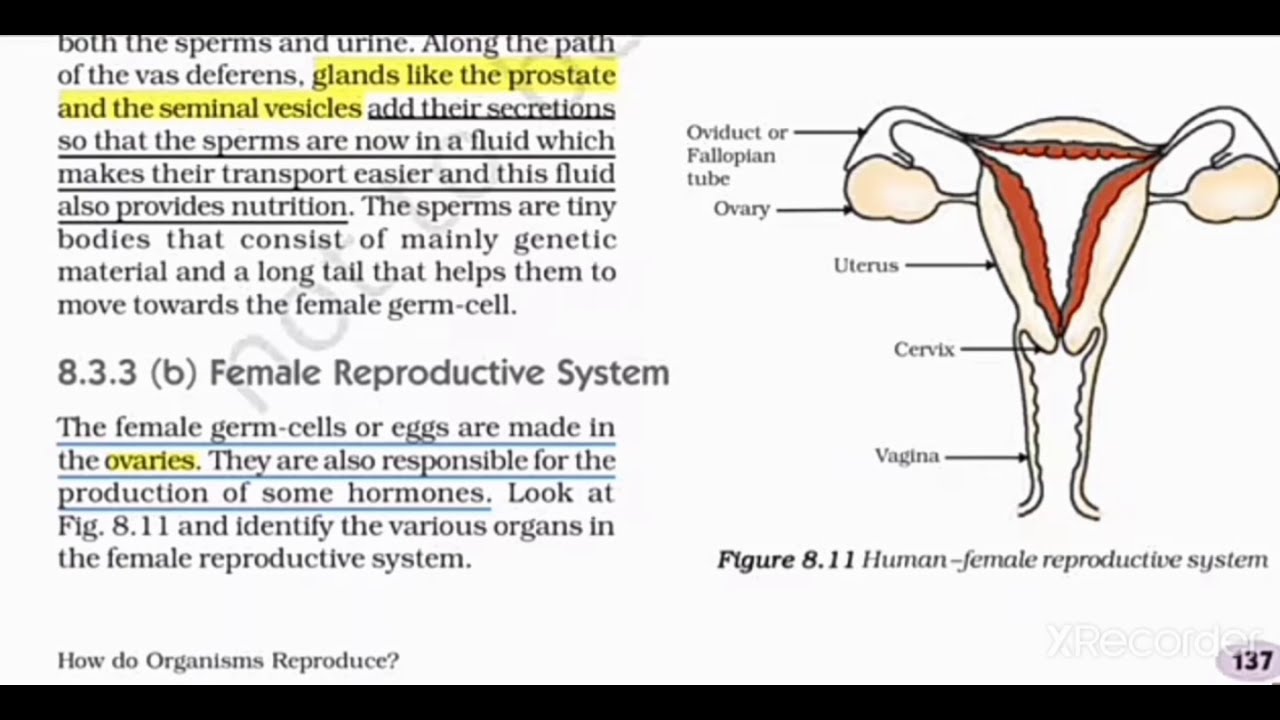The image appears to be a screenshot from a PowerPoint presentation, likely from a slide teaching anatomy. There is a black border at the top and bottom of the image, and it is labeled as slide number 137. The main content is divided into two sections: on the left is text, while on the right is an illustration labeled "Figure 8.11 Human Female Reproductive System." The illustration shows the fallopian tubes, ovaries, uterus, cervix, and vagina, with arrows pointing to each part. The text on the left discusses both male and female reproductive systems. It mentions sperms' path through the vas deferens and glands like the prostate and seminal vesicles, emphasizing how the fluid secreted aids in the transport and nutrition of sperms. It goes on to describe female germ cells or eggs' production in the ovaries, highlighting their role in hormone production. Some key terms such as "ovaries" and "glands" are underlined or highlighted in colors like white, black, yellow, blue, red, brown, and a skin-tone peach. At the bottom left, it reads "How do organisms reproduce?," alongside the text, "Section 8.3.3 Female Reproductive System." There's also a watermark at the bottom right reading "X Recorder."